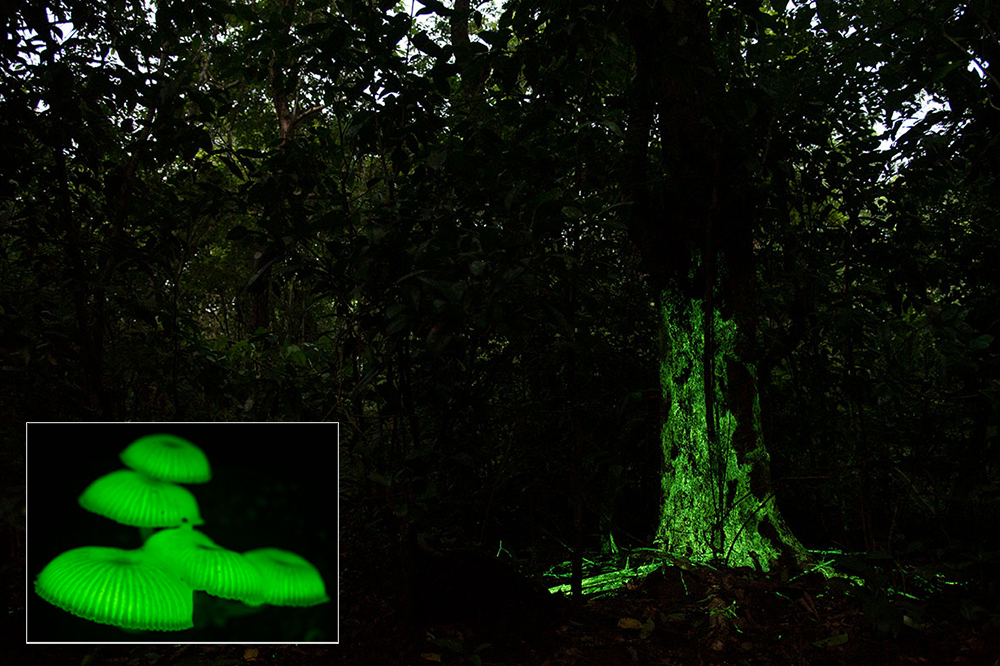The photograph appears to be taken outdoors in a dense forest during daylight, though the extensive tree cover makes it seem almost nighttime. The primary subject is a tree, dramatically illuminated by a neon green light that accentuates its trunk, extending from the roots upwards, and partially highlights its branches and leaves. In the lower left-hand corner of the image, a cluster of mushrooms shares this vibrant neon green illumination, suggesting a close-up reference to the source of the glow seen on the tree. An inset of five disc-shaped objects with curved edges and radial lines may depict these glowing fungi in greater detail. The overall scene is shrouded in darkness except for the vivid neon green, creating a contrast that focuses the viewer’s attention on the illuminated tree and mushrooms. No textual information accompanies the image to provide further context.